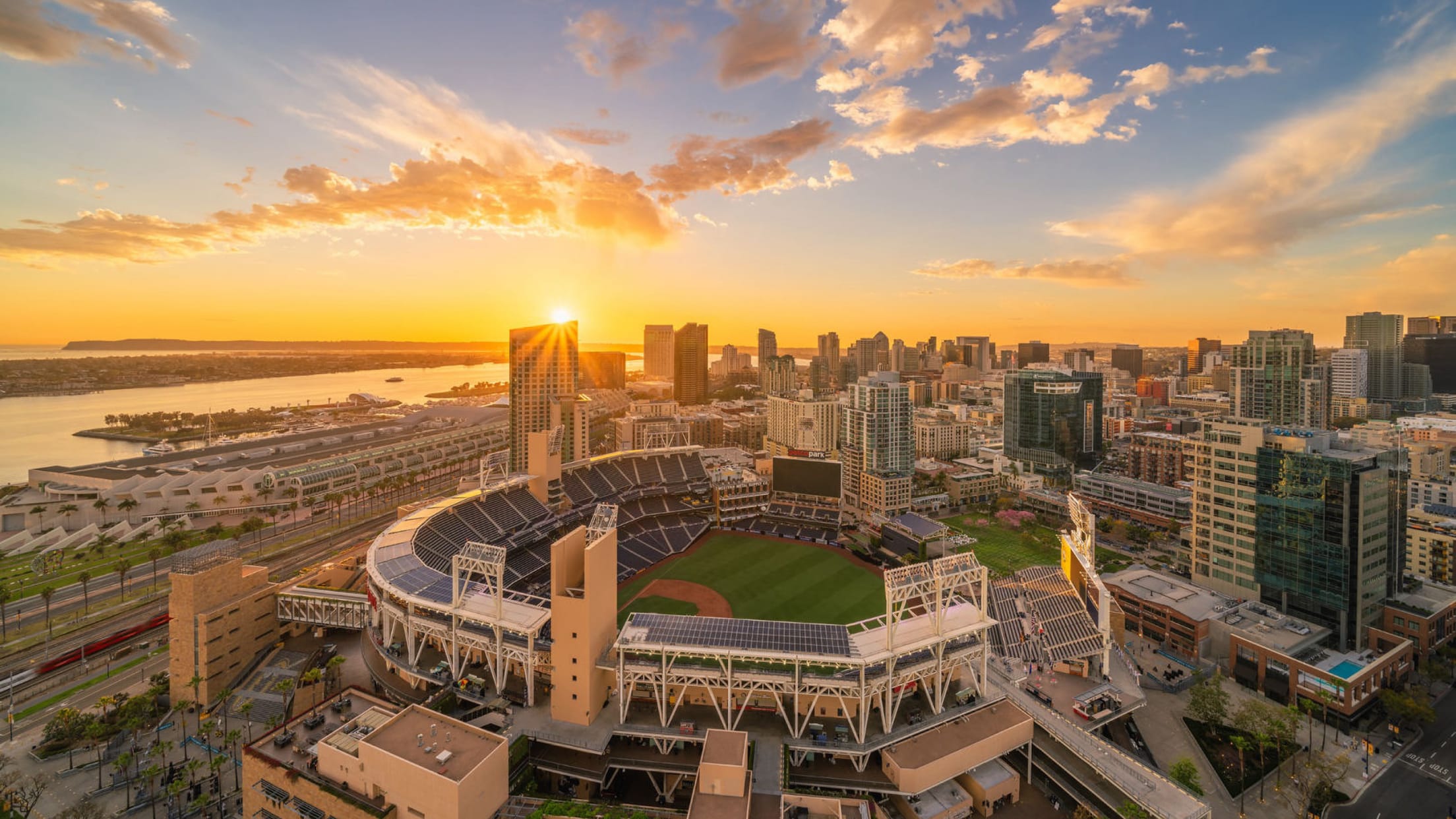This is a highly detailed, color photograph taken from an aerial perspective during the golden hour of sunset. At the center of the image is an outdoor, open baseball stadium with an empty seating area encircling a well-manicured diamond, complete with visible mow lines on the bright green grass. Surrounding the top perimeter of the stadium are solar panels. To the left of the stadium, there is a marina, its calm waters glistening under the setting sun. The background showcases a densely built city skyline, with an array of skyscrapers, some with glass facades, while others appear to be constructed from stucco and metal. The sun, a vivid bright orange, is setting behind one of the buildings, casting an orange and yellow hue across the horizon. The sky remains blue, dotted with scattered, fluffy white clouds, enhancing the vibrant contrast of the sunset. Further details include a clear view of streets lined with palm trees, adding to the scenic urban landscape.